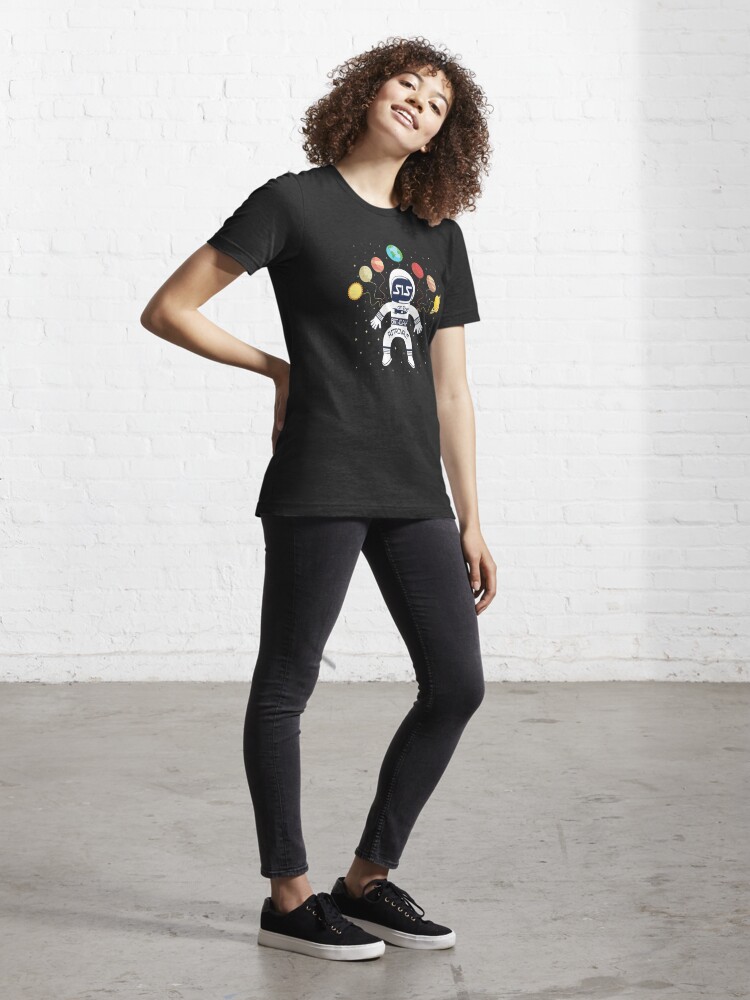In this photograph, a young black woman, appearing to be in her late teens or early 20s, stands confidently on a smooth gray concrete floor, which reflects her image. She is positioned against a white brick wall, serving as a backdrop. She has shoulder-length, curly brown hair and holds a joyful smile, her head slightly tilted back with her teeth showing. Her outfit consists of tight black slacks resembling leggings, black sneakers with white soles and no socks, and a short-sleeved, black cotton t-shirt. The shirt is adorned with a graphic featuring a central white figure resembling an astronaut surrounded by seven colorful planets in shades of yellow, tan, red, blue, and pink. Her right arm is bent at the elbow with her hand resting on her hip, while her left arm extends naturally down her side, hand against her thigh. She exudes happiness and a playful spirit.